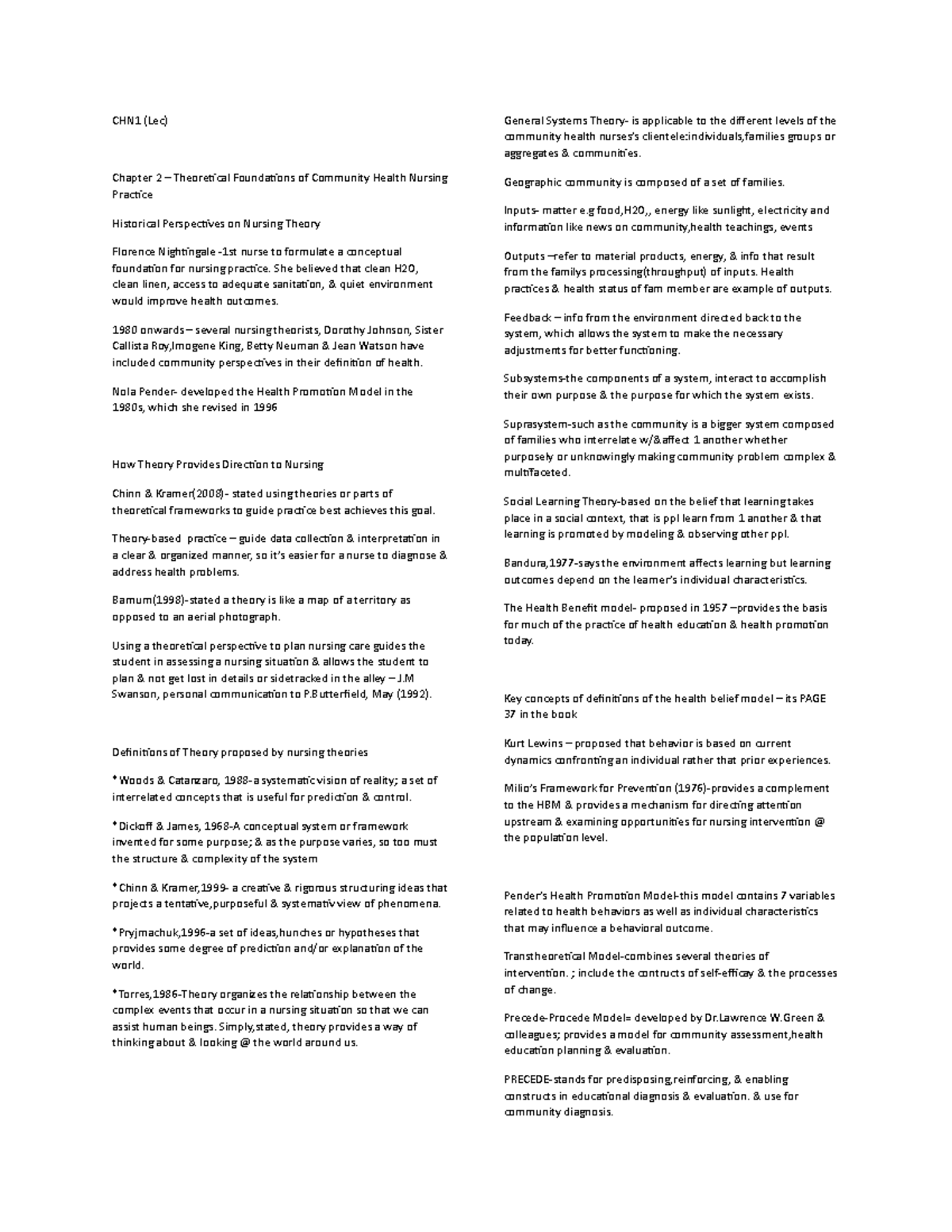The image features a plain white page with black text, bearing the header "CHN1 (LEC) Chapter 2: Theoretical Foundations of Community Health Nursing Practice." The content delves into historical perspectives on nursing theory, mentioning Florence Nightingale as the first nurse to establish a conceptual foundation for nursing practice. Nightingale emphasized the importance of clean water, clean linens, access to adequate sanitation, and a quiet environment in improving health outcomes. 

From the 1980s onwards, several nursing theorists, including Dorothy Johnson, Sister Calista Roy, Imogene King, Betty Neuman, and Jean Watson, have integrated community perspectives into their definitions of health. The health promotion model developed by Nola Pender in the 1980s, and revised in 1996, is highlighted.

The page also discusses how theory directs nursing practice. In 2008, Shannon Kramer noted that applying theories or parts of theoretical frameworks to guide practice is the most effective approach. Theory-based practice helps in the organized and clear collection and interpretation of data, facilitating the diagnosis and addressing of health problems. Additionally, Barnum in 1998 compared theory to a map of a territory rather than an aerial photograph.

The text outlines that the general systems theory is applicable to various community levels, including individuals, families, groups, aggregates, and communities, describing a geographic community as a set of families. The page contains further detailed information and a list of author's definitions and years, explaining how theory-based definitions apply to nursing practice.